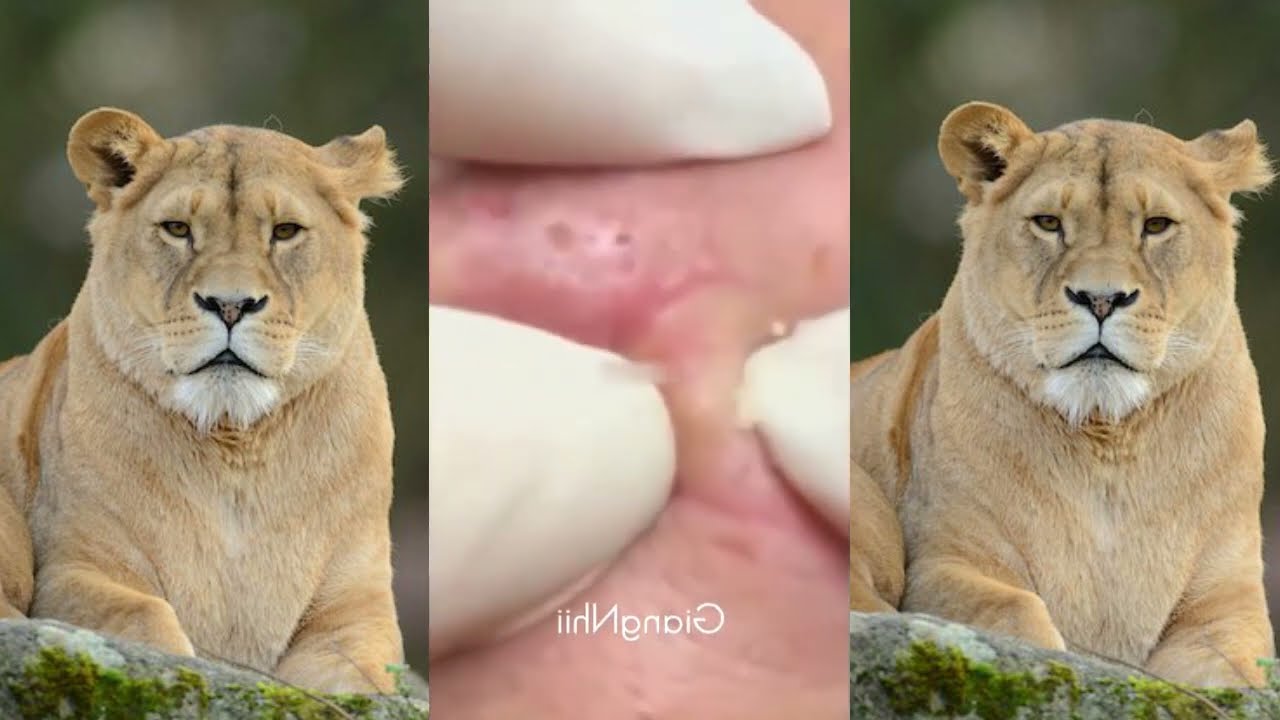The image is a wide rectangular collage consisting of three vertical photographs placed side by side. The left and right photographs are identical, depicting a lion with light yellowish-tan fur and a small amount of white fur around its mouth. The lion, which appears to be a female due to the absence of a mane, is resting on a gray stone with patches of green moss and grass at the base. The lion is looking solemnly forward, with only its front legs visible, set against a blurry green background. The central photograph features a close-up of a human hand wearing a white latex glove, pressing three fingers onto pinkish skin with purple discoloration around a white-headed acne. The fingertips, positioned in the bottom half of the image and accompanied by a finger up top for support, are in the act of squeezing the pimple.